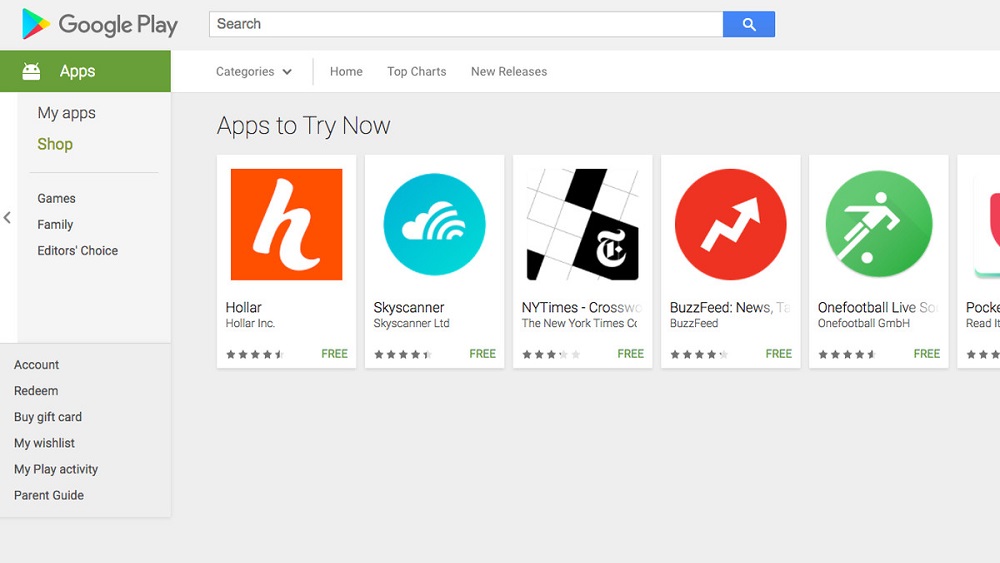This is a screenshot from the Google Play Store interface. In the upper left corner, you see the "Google Play" text, accompanied by the familiar triangular logo, all in grey. Dominating the top portion is a wide search bar featuring a blue search button.

On the left side, there's a stacked menu icon, leading to various dropdown options. Below this menu icon is the white Android head logo, signifying the app section. Directly underneath, there's a green button labeled "My Apps & Games," with "Shop" prominently displayed in green text.

A single pixel line divides this section from the content below, which includes tabs for "Games," "Family," and "Editor's Choice." Near the bottom of the screenshot, you'll find a light grey field containing account-related options such as 'Buy Gift Card,' 'My Wishlist,' 'My Play Activity,' and 'Parental Guide.'

On the right side, there are various categories including "Home," "Top Charts," "New Releases," and a segment titled "Apps to Try Now," with five featured apps partially visible. The first app is "Hollar," identifiable by a white "H" against an orange square, rated four and a half stars, and marked as free. Following this is "Skyscanner LTD," showcasing a white cloud with a beacon inside a blue circle, also free. The next app is the "New York Times Crossword Puzzle," displayed with a tilted crossword and the iconic "T," and available for free. BuzzFeed's app is represented with their logo, consisting of an arrow pointing upwards to the right. Lastly, there's "Onefootball Live" featuring a soccer player within a green circle, also free. All these app icons have drop shadows and are enclosed in green circular backgrounds.